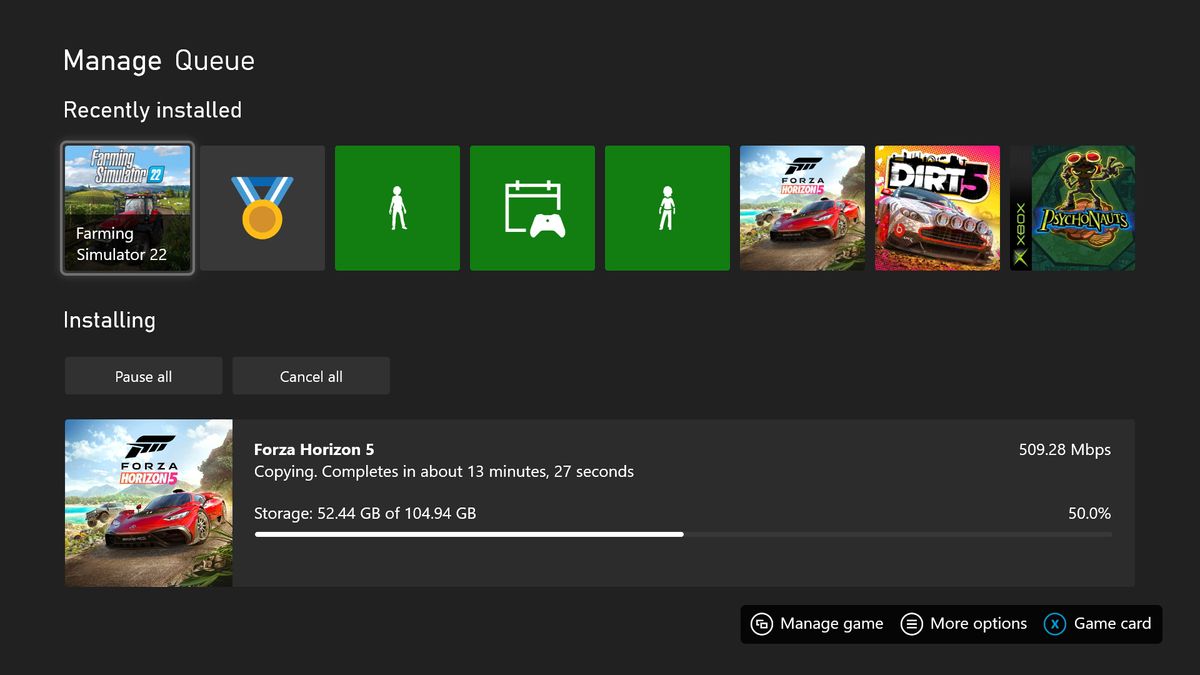This image is a screenshot from a gaming application interface displayed on a widescreen computer monitor with a dark grey background. At the top, the interface prominently features the text "Manage Queue" in white. Directly below, another line of white text indicates "Recently Installed," followed by a row of thumbnails showcasing video game covers and icons leading to different sections of the application.

The first icon in the row is for "Farming Simulator 22," depicted with a thumbnail image of a tractor on a farm. Adjacent to this is an icon of a gold medal with a blue ribbon, a green square featuring the silhouette of a person, and another green square with the silhouette of a gaming controller. Following these icons are three video game covers: "Psychonauts" for Xbox, the racing game "Forza Horizon 5," and "DIRT 5."

At the bottom of the interface, the currently installing game "Forza Horizon 5" is shown, with the data size specified as 509.28 megabytes. The estimated completion time is 13 minutes and 27 seconds. Additionally, information about the storage space is presented, showing 52.44 gigabytes used out of a total 104.94 gigabytes. A white progress bar stretches halfway across the screen, visually indicating the installation is at 50% completion.